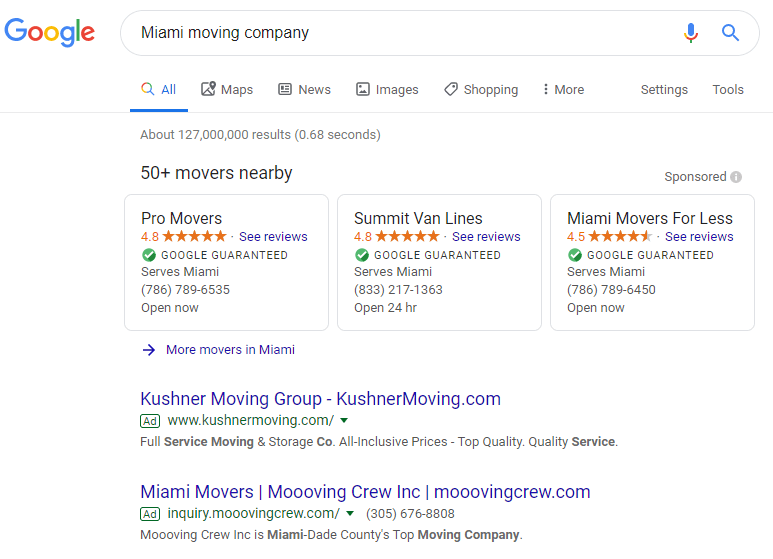The image depicts a Google search results page, characterized by the familiar Google logo in multicolored letters positioned in the top left corner. Below the logo, there is a prominently displayed search bar outlined in gray, with rounded edges at both ends, in which the query "Miami Moving Company" is entered. Flanking the search bar are icons of a microphone to the right and a magnifying glass to the left.

Directly beneath the search bar is a navigation bar highlighted by tabs, starting with "All" (underlined in blue), followed sequentially by "Maps," "News," "Images," "Shopping," and a "More" dropdown indicated by three vertical dots. Following these, "Settings" and "Tools" options also appear. 

A gray line extends below the blue underline, continuing underneath the entire navigation bar but only beneath "All" in blue. The search results indicate approximately 127,000,000 results found in 0.68 seconds. An annotated label mentions "50+ movers nearby."

On the right-hand side, there is a "Sponsored" section marked by a gray circle with an "i" inside it. This section details three moving companies:

1. **Pro Movers**:
   - Box outlined in gray.
   - Displaying orange star ratings, labeled "C Reviews" in blue.
   - A green circle with a check mark reading "Google Guaranteed."
   - Indicates the company serves Miami, provides a phone number, and shows "Open now."

2. **Summit Van Lines**:
   - Similar to Pro Movers with identical layout and features, differing only in the name.

3. **Miami Movers for Less**:
   - Displays a 4.5-star rating (slightly lower than the previous companies' ratings).
   - The section is formatted similarly to the other two.

To the right of this section is an arrow pointing right labeled "More Movers in Miami," followed by mentions of "Kushner Moving Group" displayed as "Kushner Moving Group / Kushner Moving.com."

Below these, additional ads are outlined in green, listing other moving companies such as:
- **Miami Movers**
- **Moving Crew Inc**

Each ad contains information such as a website link, phone number, and brief descriptions with black-colored text.